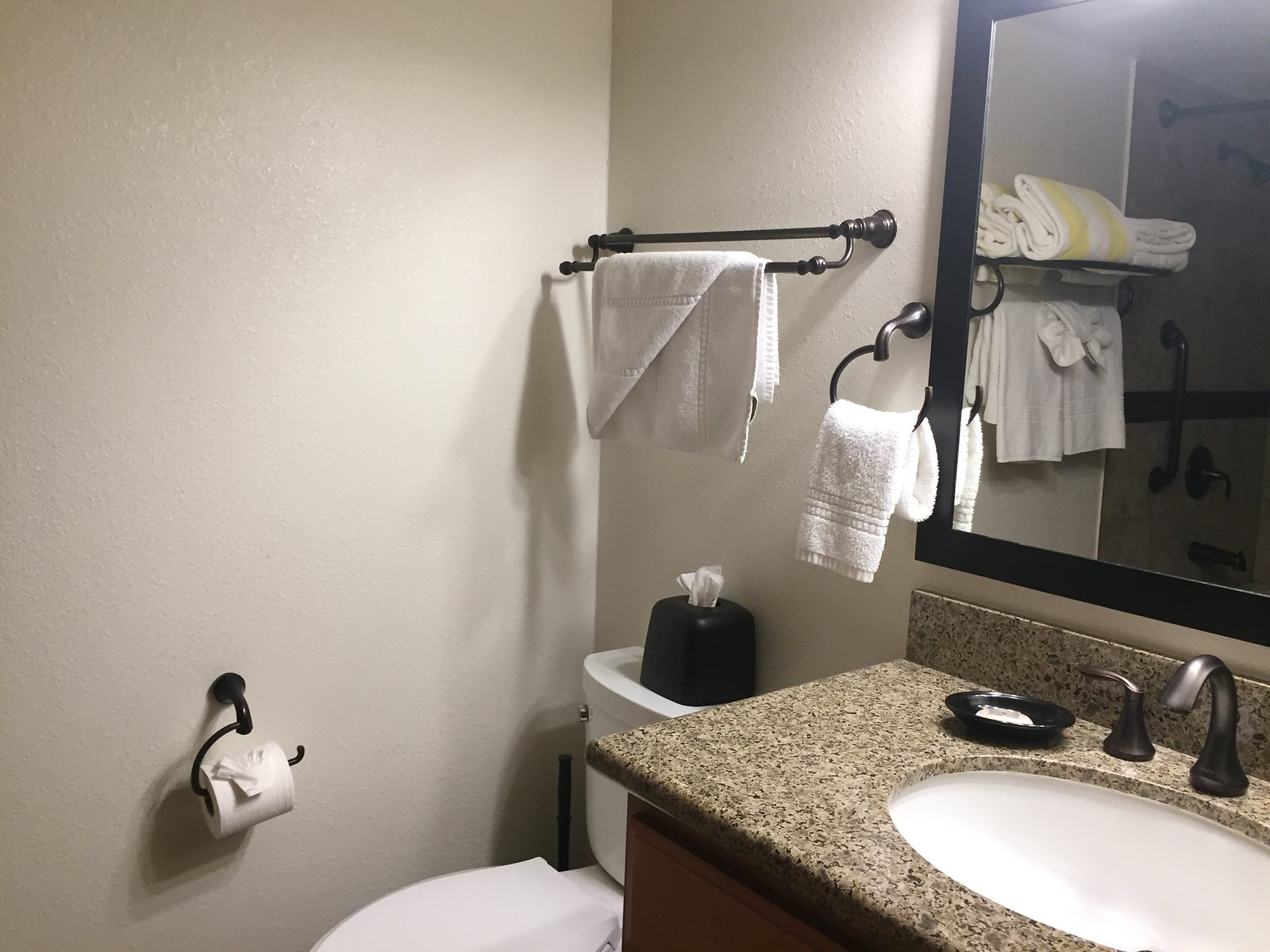This photograph captures a corner of a hotel-like bathroom decorated with light-colored walls and black accented fixtures. Prominently featured is a dark-toned wood vanity with a speckled grey granite countertop. The white porcelain sink, set within the countertop, is accompanied by faucet fixtures in a dark brushed metal finish. Above the sink hangs a rectangular mirror, framed in black, partially reflecting the rest of the bathroom.

To the right of the vanity is a white porcelain toilet, topped with a black plastic tissue holder containing white tissues. On the left wall adjacent to the toilet, a black toilet paper holder, with its roll neatly folded at the end, is mounted. In the corner next to the toilet stands a black-handled toilet brush.

Above the toilet are two towel bars, the upper one holding a wide towel, possibly a shower mat, and the lower, curved bar holding a hand towel. Both bars, like the other fixtures, exhibit a dark metal brushed finish. Reflected in the mirror, additional details can be seen, including more towels with white and yellow stripes, a handrail, a shower curtain rod, and a shower head with similarly dark brushed metal finishes.

The careful arrangement and cohesive color scheme of the black, white, and dark-toned materials contribute to the sleek and organized appearance of this bathroom.